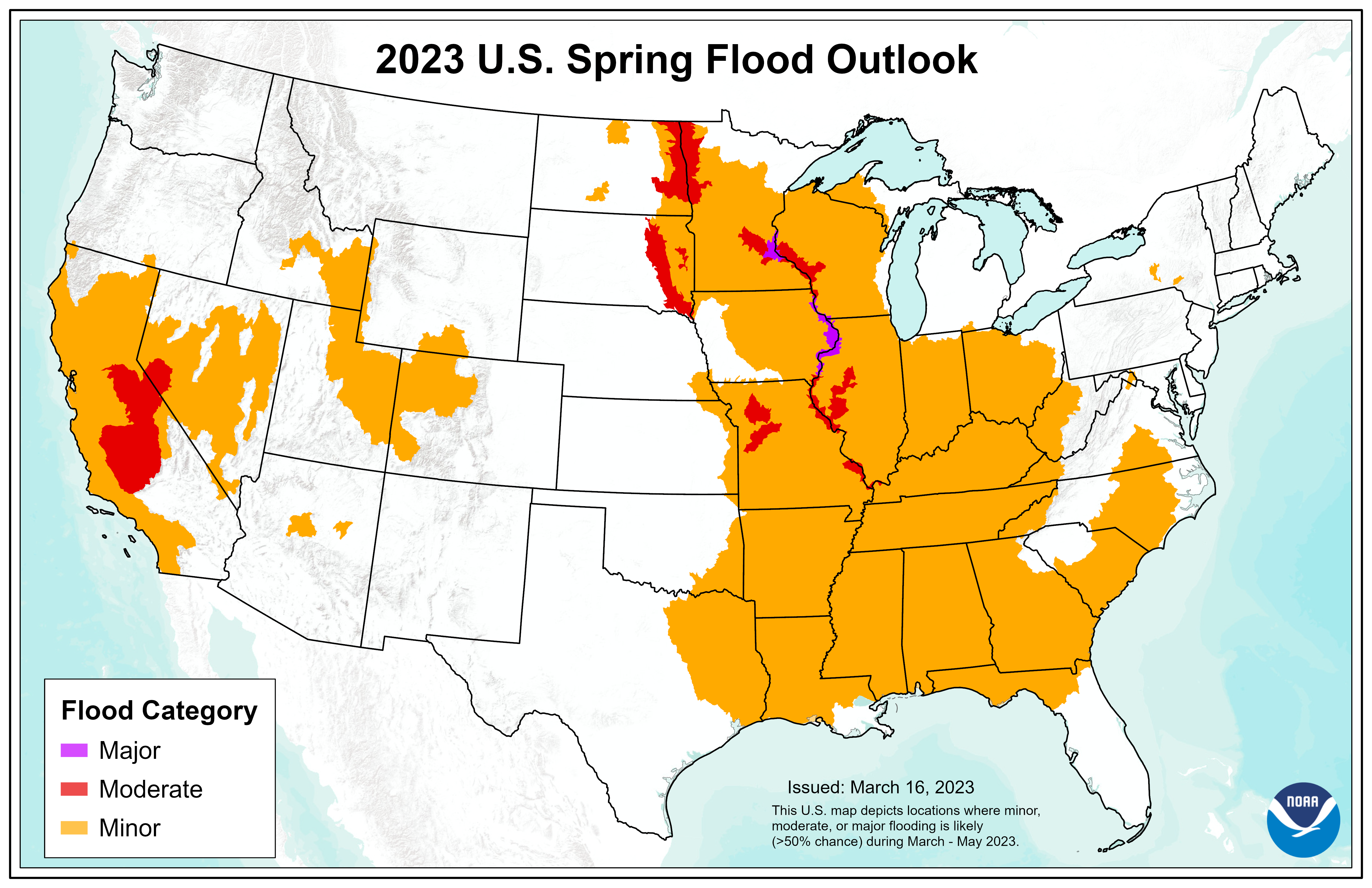This detailed image is the 2023 U.S. Spring Flood Outlook, as indicated at the top of the map. Issued on March 16, 2023, this map depicts locations with a greater than 50% chance of experiencing minor, moderate, or major flooding from March to May. The color-coded map key identifies minor flooding in tan orange, moderate flooding in red, and major flooding in purple, with areas not expecting significant flooding shown in white. 

Predominantly, most of the country is white, indicating no expected flooding. The map shows minor flooding in parts of California, Nevada, and stretches from Texas across the Southern states up to the Canadian border. California also has regions marked for moderate flooding. In the Midwest extending down to the southern United States, minor flooding is prevalent, with pockets of moderate flooding and two small areas indicating major flooding in the Wisconsin area.